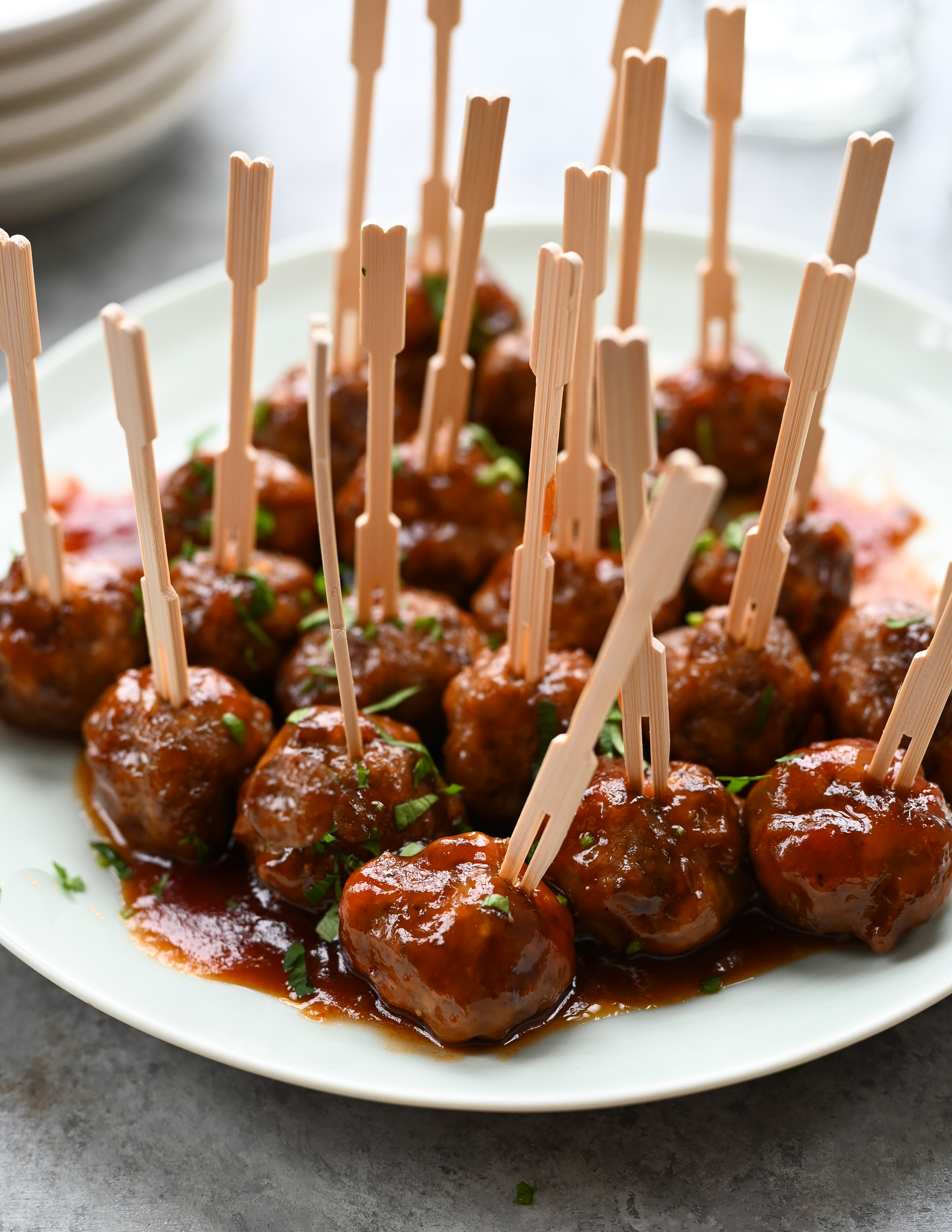This photograph captures a white plate brimming with dark brown teriyaki meatballs, each skewer adorned with a unique, light beige fork-shaped toothpick for easy handling. The meatballs are richly coated in a glossy, reddish-brown teriyaki glaze that pools slightly at the bottom of the plate, enhancing their savory appearance. Fresh, vibrant green parsley is sprinkled atop, adding a pop of color and a hint of freshness to the dish. The plate is centrally placed against a dark gray, granite-like surface, offering a contrasting backdrop that emphasizes the delectable visual appeal of the meatballs.